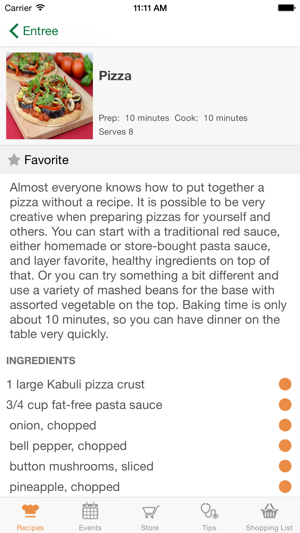**Caption:**

A user’s cell phone screen displays a detailed pizza recipe page. At the very top, the screen shows standard status bar elements: "carrier" on the left with a sound wave icon, the time “11:11 a.m.” in the center, and a full battery icon on the right, all in black on a white background.

Just below, the interface indicates the category with “ENTREE” in green text, flanked by a green back arrow on the left. The user is viewing a section dedicated to entrees.

A horizontal rectangular gray box lies below, featuring an appetizing photo of two freshly cooked pizzas on a wooden cutting board with tomatoes in the background on the left. To the right of the photo, the bold black text reads “Pizza.” Beneath this, in lighter gray text, it specifies: “Prep: 10 minutes, Cook: 10 minutes, Serves: 8.”

Directly under the preparation details, a darker gray ribbon with a gray star icon on the left reads "FAVORITE" in black text, indicating the option to favorite the recipe.

A descriptive paragraph in gray text follows, highlighting the versatility and quick preparation of making homemade pizza. It explains the creative freedom in choosing ingredients, whether using traditional red sauce or experimenting with mashed beans and assorted vegetables, emphasizing the short baking time of 10 minutes.

Below the description, the word “INGREDIENTS” appears in bold, gray, all-capital letters, introducing a list of necessary ingredients. Each ingredient is marked with an orange filled-in circle on the right.

At the bottom of the screen, a light gray navigation bar presents several icons for different sections: "Recipes," "Events," "Store," "Tips," and "Shopping List." The "Recipes" icon is highlighted in orange, matching the orange dots alongside the ingredients, indicating that the user is currently in the recipes section. 

This detailed recipe page provides all the essential information for creating a delicious homemade pizza efficiently.